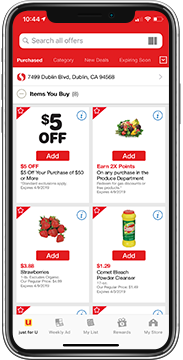This image, captured from a cell phone, showcases a screenshot of a shopping app. The interface displays a series of grocery items that the user can add to their cart. At the top right corner, the time is shown, reading 10:44. Several icons are also visible, including the battery indicator, which appears to be at approximately 30%. 

Directly below these indicators is a search bar with a magnifying glass icon, labeled "Search All Offers." At the far right end of the search bar, there is a barcode icon. The user has selected the "Purchased" tab, which has brought up a list titled "Items You Buy" followed by a number in parentheses indicating the quantity.

Below this, the user's address is displayed, located on Dublin Boulevard in Dublin, California, along with their zip code. The current view displays four items on the visible part of the screen, with the possibility of viewing two additional items by scrolling, suggesting the presence of more items in the list.

A prominent $5 off coupon is featured at the top of the food list, which can be added to the cart. From the produce department, there is an option to add products and earn 2% rewards points. The visible items in this section include strawberries and Comet bleach powder cleaner.

The detailed layout and options indicate a user-friendly shopping experience, emphasizing both convenience and efficiency.